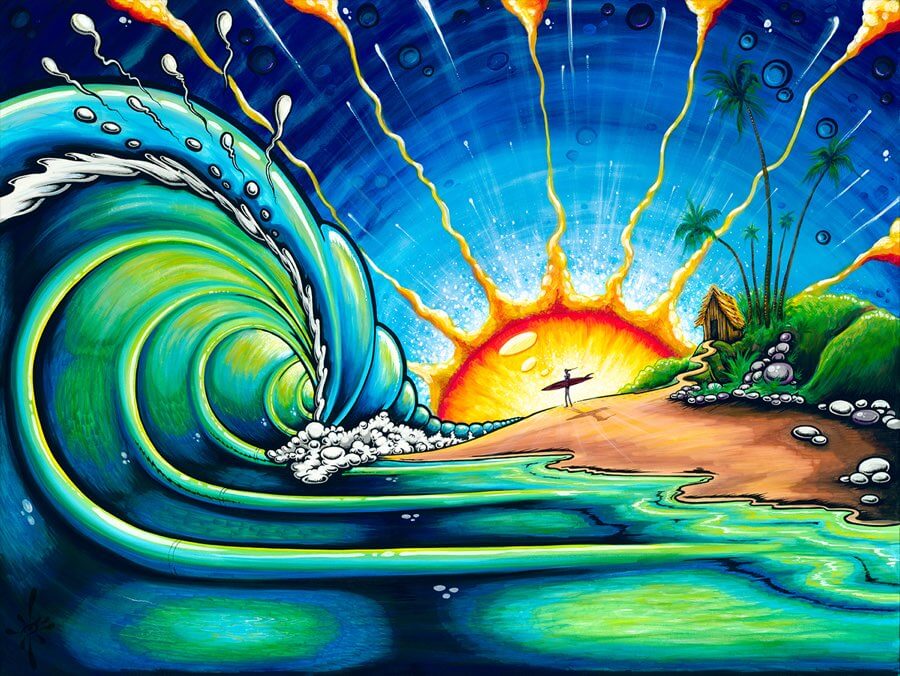The image is an abstract painting of a beach scene featuring a lone surfer heading towards an immense, curling wave. The wave, which exhibits a striking greenish-blue gradient, appears almost alive with droplets of water depicted as flying sperm. The surfer, carrying a surfboard, is depicted in the middle ground, advancing towards the tumultuous sea. Above, the sun shines prominently, its rays spreading outward, creating a dramatic backdrop. To the left of the scene, perched atop a grassy hill, is a small cabin-like structure with a sandy trail leading up to it, flanked by silver rocks and sporadic palm trees. The beach stretches from the middle to the right side of the painting, where the wave’s curling motion culminates into a splash against the shore. The overall color palette includes variations of yellow, aqua, light blue, and dark blue, with the surreal elements conveying a vivid and dynamic coastal atmosphere.